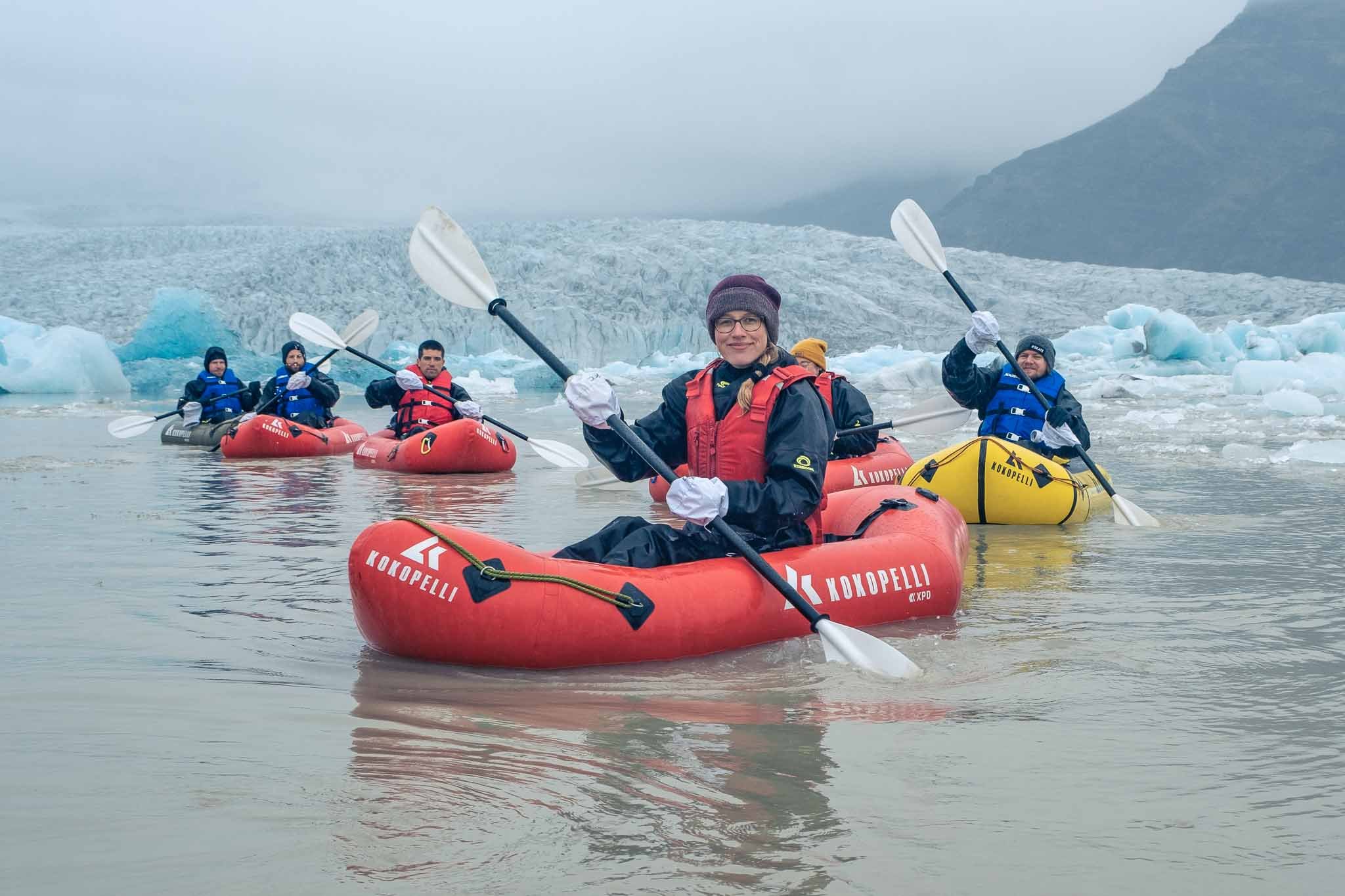In this evocative landscape photograph, a group of six kayakers navigates an icy Arctic waterway filled with scattered icebergs. Dominating the foreground is a smiling woman in a red inflatable kayak, dressed in a dark black suit and red life preserver. She is equipped with white specialized mittens, black oars with white paddles, and a dark purple beanie covering her braided hair. She also wears glasses, her expression one of enjoyment and adventure. Moving further into the photo, a second kayaker in a yellow inflatable kayak and blue life jacket is slightly to her right, while directly behind her, another red inflatable kayak partially obscures its occupant. Flanking these central figures, there are two men in blue life jackets, both with facial hair, and another person in a gray inflatable kayak, all set against a misty backdrop of snow-covered mountains and a gray sky. The scene is a striking interplay of vibrant kayak colors—four red, one yellow, and one gray—against the muted tones of the Arctic landscape. The water, still and almost reflective, mirrors the serene and frigid beauty of their expedition.